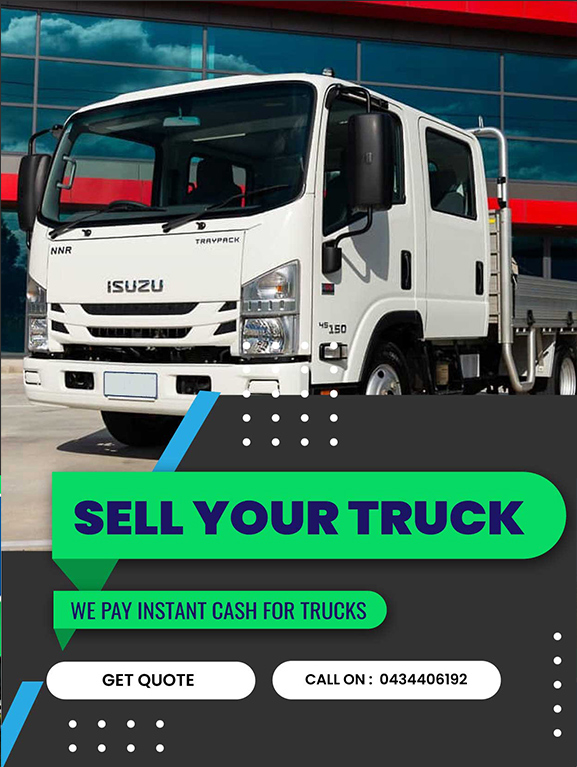This image is a cropped screenshot from a commercial website. Dominating the top section of the image, there's a clear picture of a white ISUZU truck facing forward, with its cargo area open and painted in grey. The truck is parked in front of a large office building that features a windowed façade with red accent panels at the top and bottom. The reflective glass windows capture the cloudy sky above. 

The ground beneath the truck appears to be a smooth, grey surface. Scattered across the image are some white dots forming a pattern, with several appearing to the lower left and a vertical formation of five dots toward the lower right.

A black background section, angled diagonally across the middle of the image, separates the top visual from the text and advertisements below. On this black strip, there's a prominent green rectangle with a curved right edge, containing the text, "Sell your truck," written in blue. Below that, a smaller green rectangle, also with a curved right edge and tucked partially behind the black background, reads, "We pay instant cash for trucks."

Further down, a white rectangular button with rounded edges says, "Get a quote," and within this button, there's a call to action with the contact number "Call on 0434405192." Overlaying this section are additional design elements comprising blue diagonal bands framing the green rectangles, with breaks aligning with the placement of these green elements.